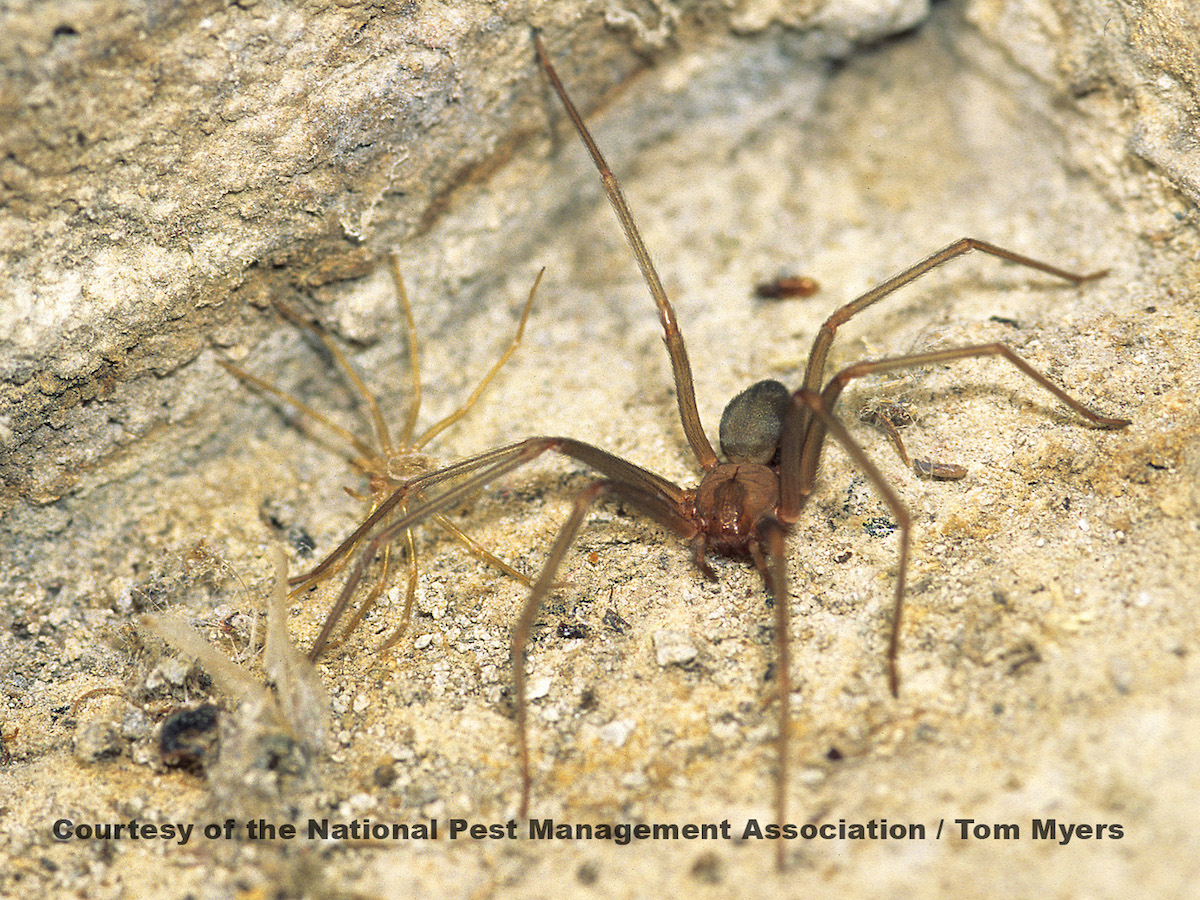This photograph features two distinctive brown recluse spiders on a large boulder. Dominating the scene, the larger spider exhibits long, brown legs with a darker brown or black body, marked by a prominent violin-shaped pattern stretching from its eyes down its back. To the left, a smaller, lighter-colored spider, possibly a juvenile due to its size and slightly golden hue, shares the boulder. They both rest on the rocks amid scattered rock fragments, adding texture to the sandy, tan ground around them. The image includes a caption at the bottom, stating "Courtesy of the National Pest Association / Tom Myers," presented in black font. The photograph captures the intricate and somewhat unsettling details of these spiders, highlighting their striking size and hallmark features.